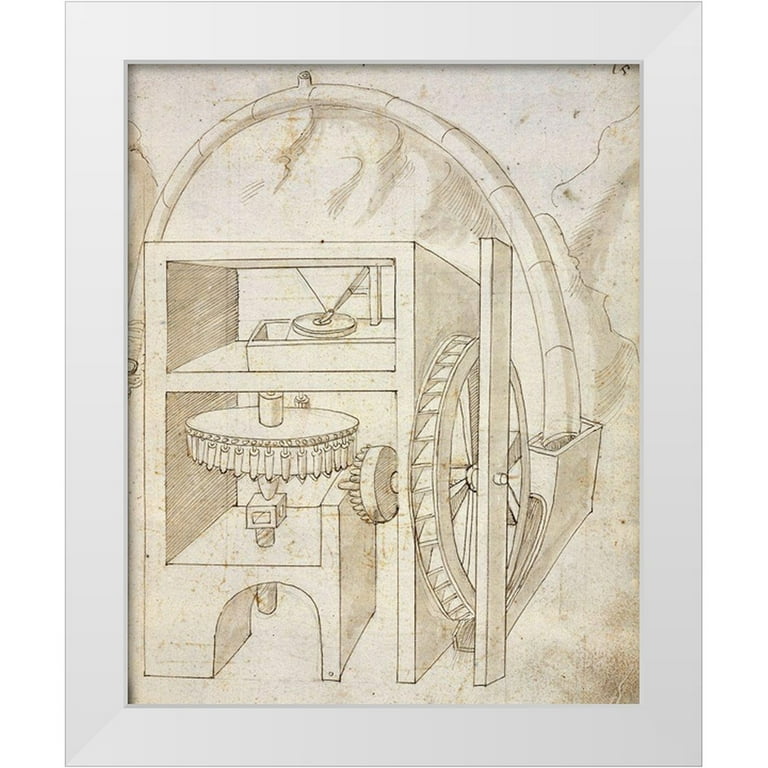This detailed pencil sketch illustrates the inner workings of a complex machine, housed within a box frame. At the center of the machinery is a large gear that closely resembles a water wheel, distinguishable by its substantial size compared to the smaller, interlocking gears inside the box. This large gear appears to have a long board attached to it, possibly allowing it to be spun manually. The smaller gears within the framework are arranged in both horizontal and vertical orientations, engaging with each other to create a synchronized, clockwork-like motion. Notably, there is a rectangular piece inside the box with a circular part that seems to spin continuously, adding to the intricate mechanical operation. Outside the main gear system, a large pipe-like device extends from just beyond the wheel, arches over the top of the structure, and disappears off the left side of the image, hinting at a more complex mechanism at play. The entire scene is drawn in a classical style, resembling an old black-and-white sketch, set against a backdrop of what appear to be marble walls and flooring, suggesting a historically significant or aesthetically sophisticated environment.